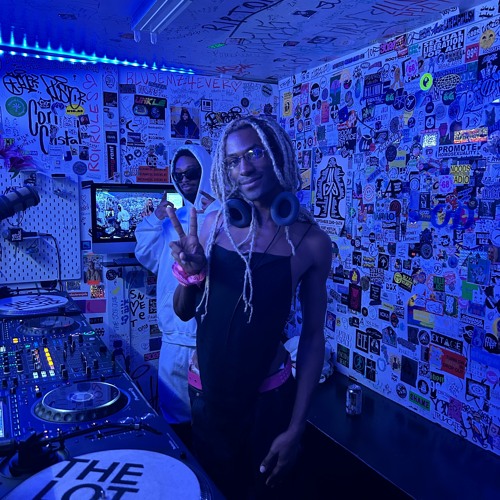In a dimly lit room with a blue neon glow, two DJs are captured posing for the camera against a backdrop of graffiti-like artwork, labels, and colorful posters covering the walls and ceiling. The room is filled with an array of DJ equipment, including turntables, records, buttons, and yellow lights flashing on a black DJ desk. 

The main person in the forefront, showcasing a peace sign with their right hand, has long blonde-dyed braids, a darker complexion, and clear eyeglasses. They are wearing black headphones around their neck, a black tank top with open armholes, black pants, and a pink belt. Beside them stands another individual in a white hoodie and white shorts, wearing dark sunglasses and holding up a thumbs-up sign. 

Amid the eclectic decor and artistic chaos, a television mounted on a stand can be seen in the background, adding to the vibrant ambiance of the scene.